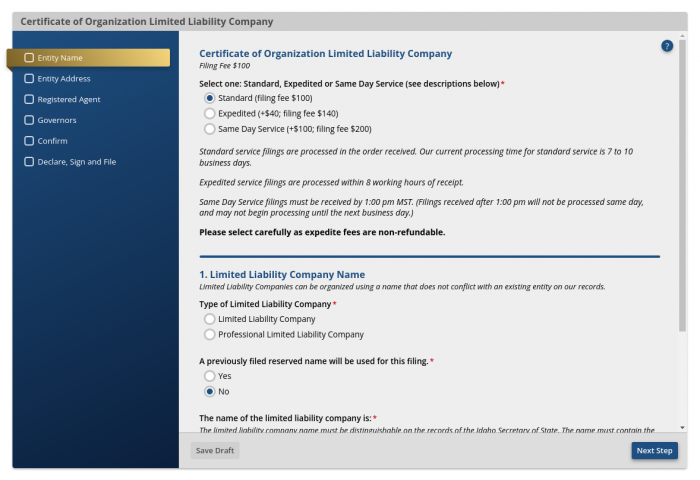The website for Certificate of Organization Limited Liability Company provides a streamlined process for filing business documents. At the top of the website, the company's name is prominently displayed in gray, followed by a repetition in blue. The filing fee is clearly stated as $100.

Users have the option to select from three service types: standard, expedited, or same day delivery. A red asterisk marks required fields and additional important information. The standard service, selected by the user, has a $100 filing fee and standard service filings are processed in the order they are received, with a current processing time of 7 to 10 business days.

Expedited service is processed within 8 working hours, and same day service requires receipt by 1 p.m. MST, with any submissions after that time starting processing the next business day. Users are cautioned to choose carefully, as expedite fees are non-refundable.

For the filing process, users can select a Limited Liability Company or Professional Limited Liability Company, and indicate if a previously filed reserve name will be used. Step-by-step prompts guide users through necessary fields like entity name, entity address, registered agent, governors, confirmation, declaration, signing, and filing. 

A navy blue column on the left side of the page contains checkboxes for each step, ensuring a clear, organized process for completing the filing.